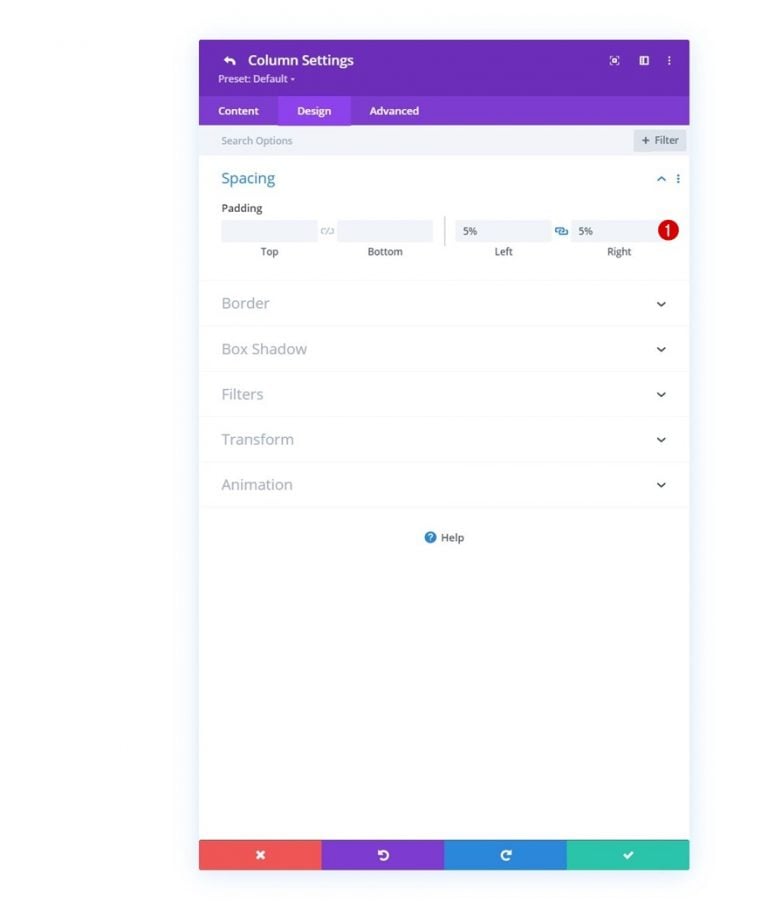This is a detailed screenshot of a mobile app's settings menu. At the top, there's a prominent purple bar. In the upper left corner of this bar, a white arrow points left, and next to it, "Column Settings" is written in white font. Below, "Preset: Default" is displayed, accompanied by a downward-pointing white arrow. On the upper right corner, there are three icons—a screenshot icon, a minimize icon, and a menu icon consisting of three vertical white dots.

Beneath the purple bar is a lighter purple bar, also featuring text in white font. It reads "Content Design" with sections "Content" and "Advanced" grayed out while "Design" is selected. Below this, a white page occupies most of the screen.

At the top of the white page, "Search Options" is indicated. In the upper right corner, there's a gray button labeled "Plus Filter." Below this, in gray font, is the word "Spacing," followed by text fields labeled "Padding: Top, Bottom, Left, Right." The values in the "Left" and "Right" fields are both set to "5%."

Further below, there are several drop-down menus labeled "Border," "Box Shadow," "Filters," "Transform," and "Animation." At the bottom of the screen, there is a small blue circle with a white question mark inside it, accompanied by the word "How."